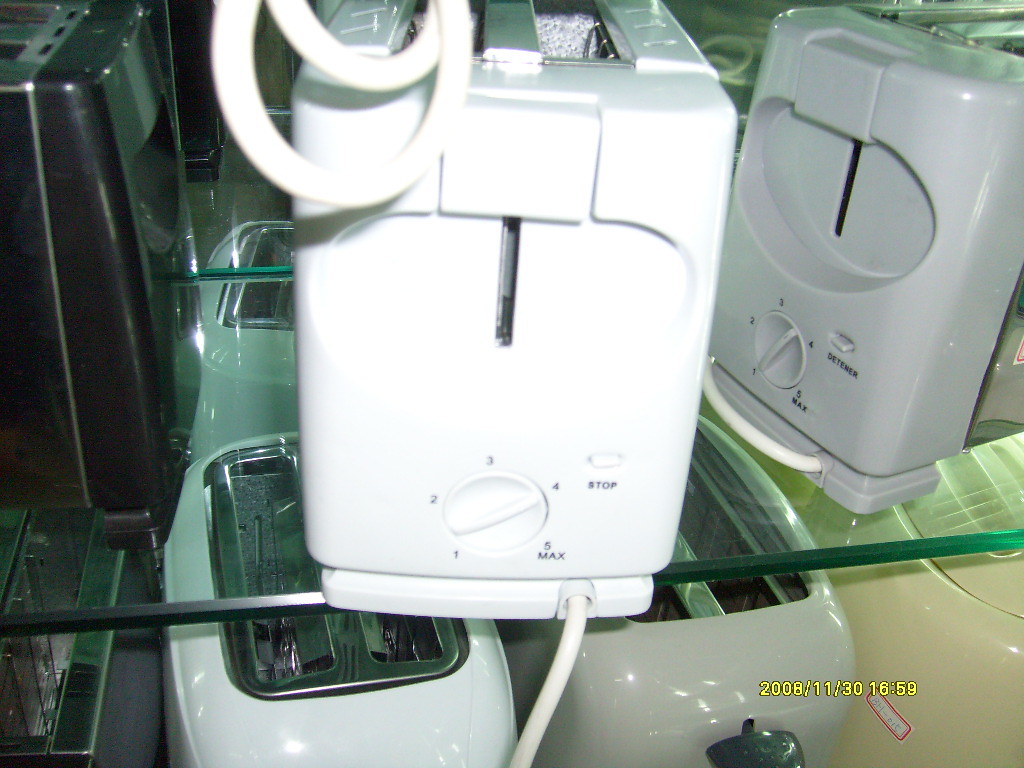This image is a low-quality color photograph of several toasters arranged on glass shelving, likely in a store, repair shop, or pawn shop. The central focus is a white toaster with a coiled white cord, prominently displayed on a top glass shelf with a light green edge. Next to it is an off-white toaster, and a black and silver toaster is visible on the left side. Below the glass shelf, additional toasters in a variety of colors—including gray, cream, yellow, beige, and black—are seen, positioned on another shelf beneath. These toasters feature a front knob labeled from 1 to 5 with "Max" under 5 and a "Stop" button to the right. The lighting creates reflections and highlights on the toasters' surfaces. The lower right-hand corner of the image is stamped with the date "2008-11-30" and the time "16:59." The toasters appear to have a typical two-slot design with curved sides leading to their open tops.